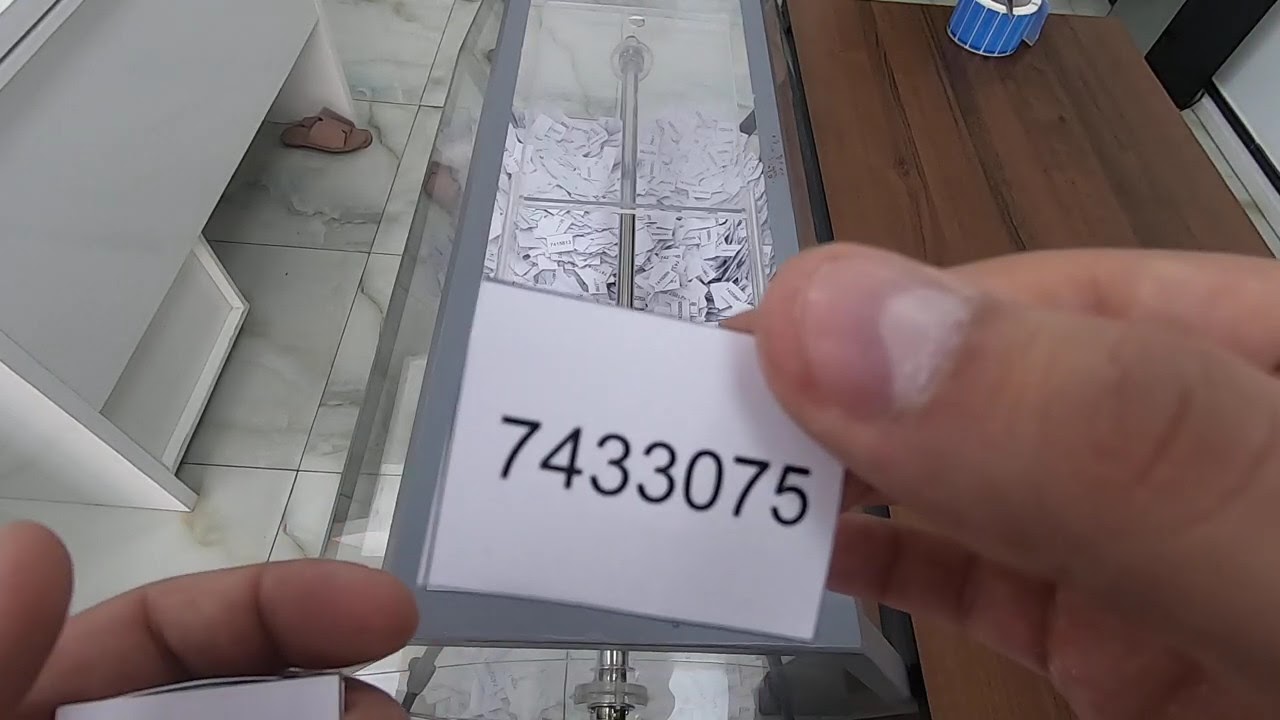The photograph captures a pair of medium brown hands, with noticeably short fingernails, holding up a white rectangular piece of paper between the thumb and index finger. The slip of paper features the printed number "7433075" in black text. The hands appear above a glass cabinet filled with numerous other similar numbered slips. To the right of the glass cabinet, there is a medium-toned wooden bench with a roll of blue stickers on it. To the left, a white desk stands over a white and slate gray patterned tiled floor, under which lies a lone tannish-mauve sandal. A pipe runs across the bottom of the image, adding to the scene that suggests this is an environment like a shop or store, possibly preparing for a raffle or lottery event.